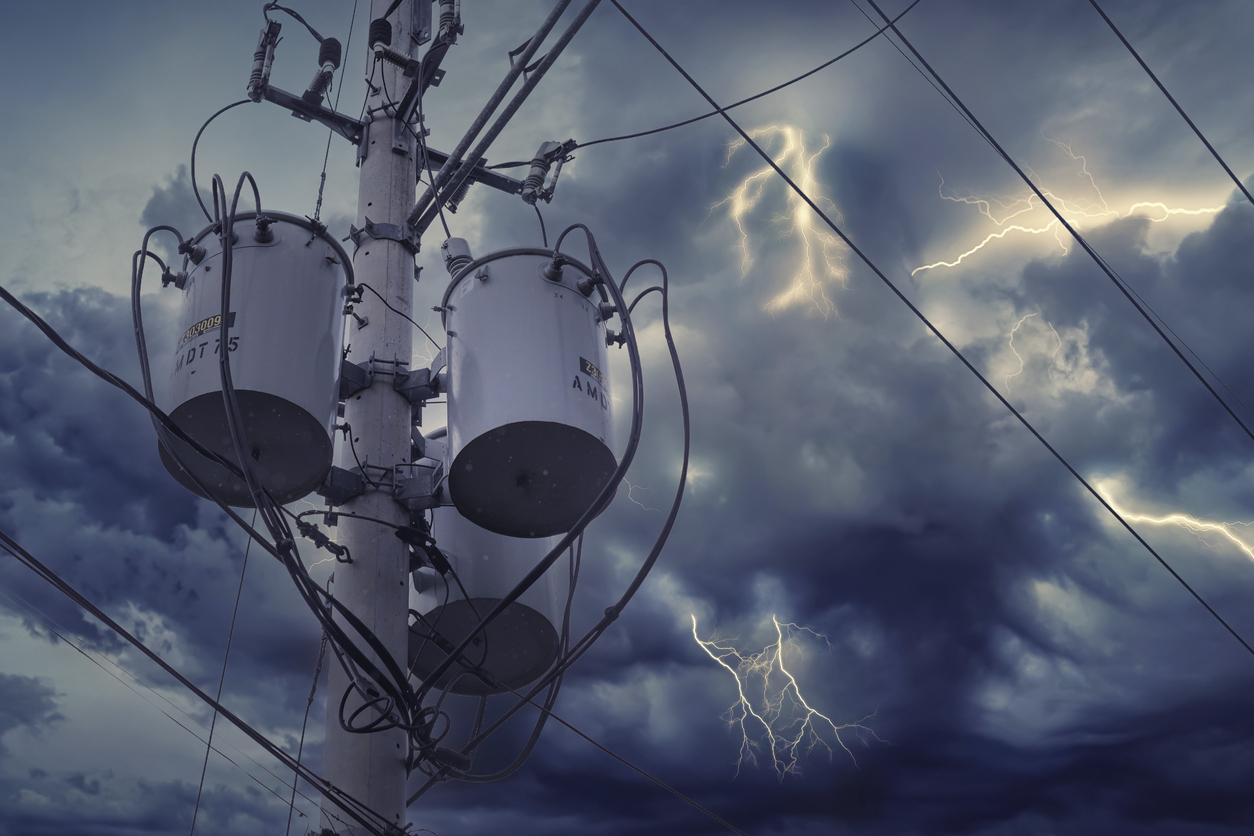The photograph captures a dramatic and stormy sky, teeming with dark grayish-blue clouds and streaked by multiple lightning bolts. The viewer's gaze is drawn upwards, from the ground, emphasizing the imposing height of the high voltage utility pole that dominates the left side of the image. This towering metal structure is adorned with three large, cylindrical canister-like transformers labeled "MDT75," from which a web of wires and cables emanate. These cables crisscross diagonally across the image, intersecting with dark, turbulent clouds that form the backdrop. The photograph reveals three distinct lightning strikes: one near the middle top-right, another slightly closer to the right edge, and a final bolt piercing the bottom middle portion of the canvas. The scene is an intricate interplay of man-made and natural elements, capturing the raw power of the storm and the sturdy resilience of the electrical infrastructure amidst the chaos.